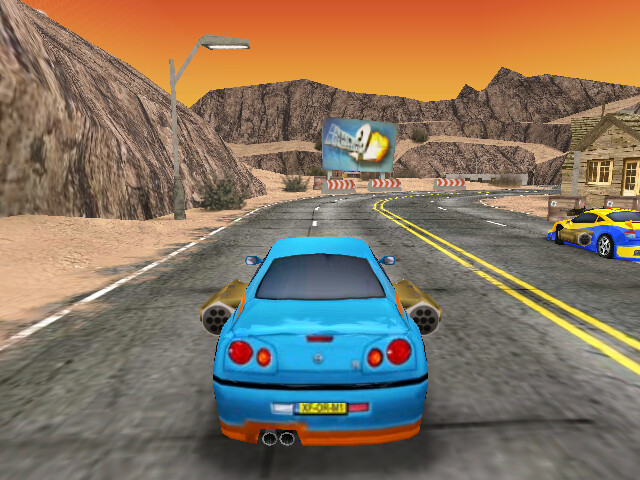This image appears to be a screenshot from an older racing video game, likely from the PlayStation 1 or PlayStation 2 era, based on the graphical quality. The scene is set in a desert town featuring a rounded road with two lanes separated by a double yellow line. In the foreground, there is a prominent blue car with an orange bumper and distinct rear lights—one red and one smaller circle beside it—indicating it's the player-controlled vehicle. The blue car appears to be equipped with helicopter gatling guns mounted along both sides, suggesting this is a combat racing game. On the right side of the image, there is another car, presumably an opponent, positioned slightly ahead on the road. The road is bordered by a small structure, possibly an old cabin, emphasizing the rustic setting. Notably, the image seems to be cropped or zoomed in, as there are no visible UI elements, which could also indicate it was edited for advertising purposes.